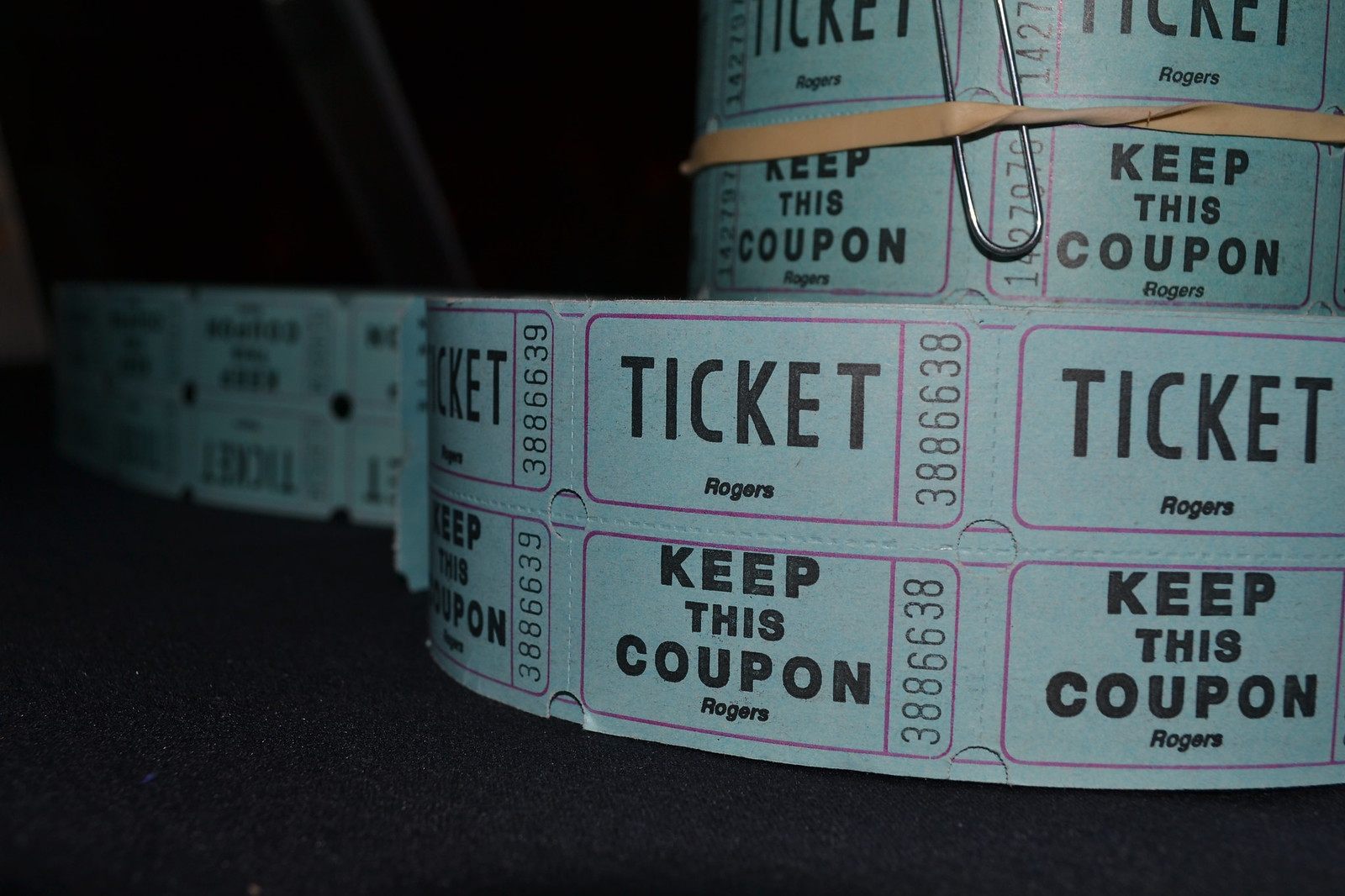This photograph showcases a dramatic scene of vintage-style blue tickets against a pure black background, emphasizing their nostalgic flair. Dominating the right side, a large bottom roll of tickets spools outward and stretches into the darkness, creating a sense of elongated depth as it fades to the left. Positioned neatly atop this large roll is a smaller roll, secured with a rubber band and an additional paper clip for support. The tickets are meticulously detailed, displaying sequential numbers such as 388-6639, 388-6638, and 1427978. Each ticket reads "Ticket" and "Keep This Coupon," with a mention of "Rogers," and they are outlined in pink, adding a delicate contrast to their soft gray hue. The entire composition is shrouded in mystery, as the surrounding blackness leaves one guessing the context of the scene.